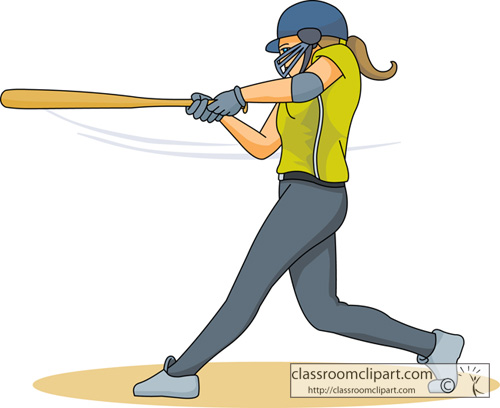This clip art image, created by classroomclipart.com, features a cartoon depiction of a young softball or baseball player in mid-swing. The player, a girl with brown hair pulled back in a ponytail secured by a yellow hair tie, is shown standing in a circle of dirt. She is wearing a blue batting helmet with a face guard, and blue batting gloves. Her outfit consists of a yellow short-sleeve jersey with a white pinstripe and blue stripe on the edge underneath her arm, along with gray-blue uniform pants and gray sneakers.

The girl is depicted with her bat extended out in front of her, both hands gripping it firmly. She is adorned with gray elbow pads and a black undershirt beneath her uniform. The bat is shown with swoosh lines trailing behind, indicating that it was recently swung. Details of the image include textual annotations at the bottom right corner, reading "classroomclipart.com" and "http://classroomclipart.com."